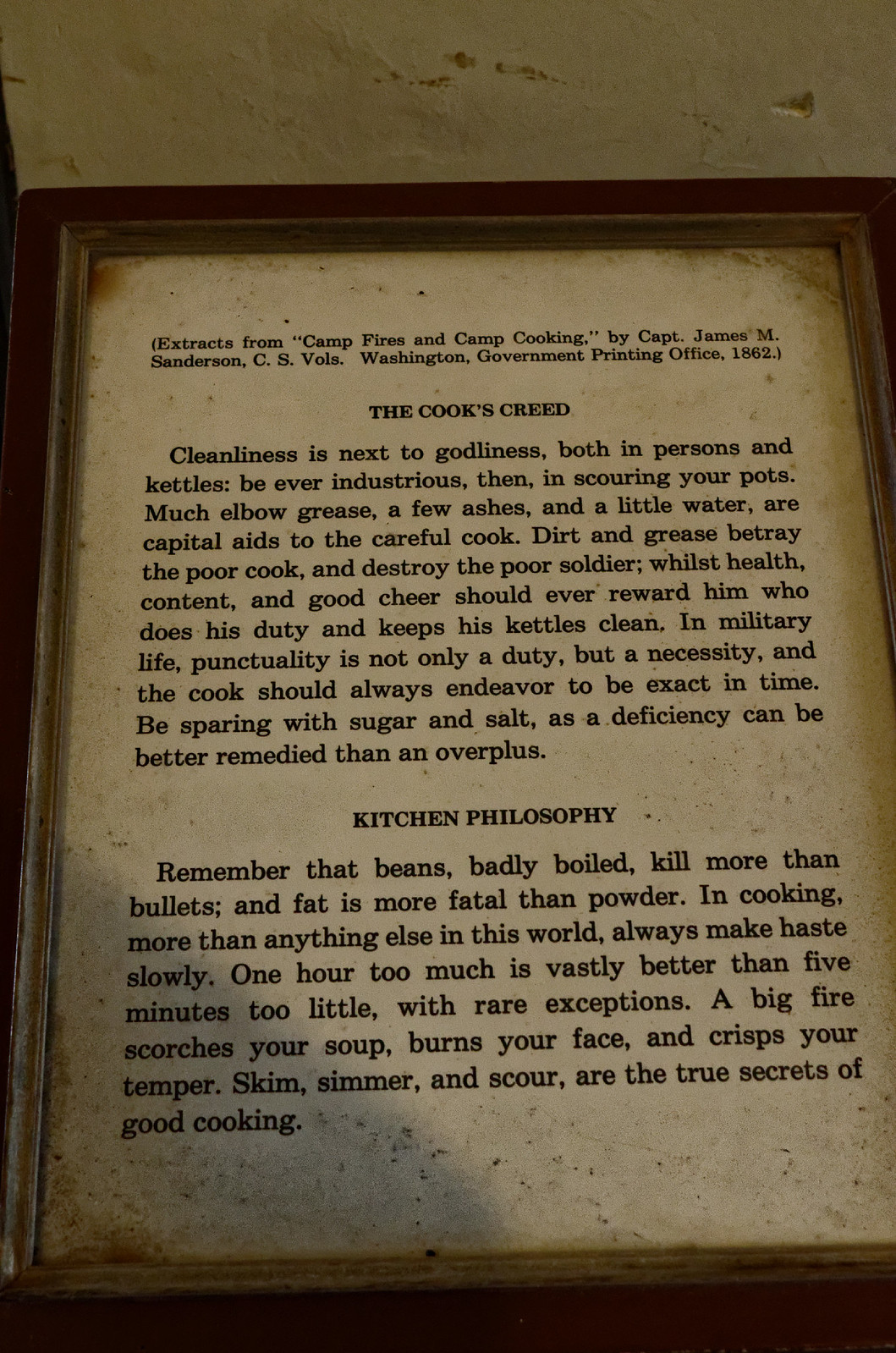This image depicts an aged, creamy white page framed in wood, likely on display in a museum or collection. The text is a historical excerpt titled "Extracts from Campfires and Camp Cooking" by Captain James M. Sanderson, C.S. Valls, published by the Washington Government Printing Office in 1862. The page is divided into two sections. The first, "The Cook’s Creed," extolls the virtues of cleanliness: "Cleanliness is next to godliness, both in persons and kettles. Be ever industrious, then, in scouring your pots. Much elbow grease, a few ashes, and a little water are capital aids to the careful cook. Dirt and grease betray the poor cook and destroy the poor soldier, while health, content, and good cheer should ever reward him who does his duty and keeps his kettles clean." It further advises on the importance of punctuality and a judicious use of sugar and salt, noting that "a deficiency can be better remedied than an overplus." The second section, "Kitchen Philosophy," offers practical and philosophical cooking advice: "Remember that beans, badly boiled, kill more than bullets, and fat is more fatal than powder. In cooking, more than anything else in this world, always make haste slowly. One hour too much is vastly better than five minutes too little, with rare exceptions. A big fire scorches your soup, burns your face, and crisps your temper. Skim, simmer, and scour are the true secrets of good cooking." The text emphasizes both the practicality and the philosophical approach to camp cooking, making it a valuable piece of culinary history.